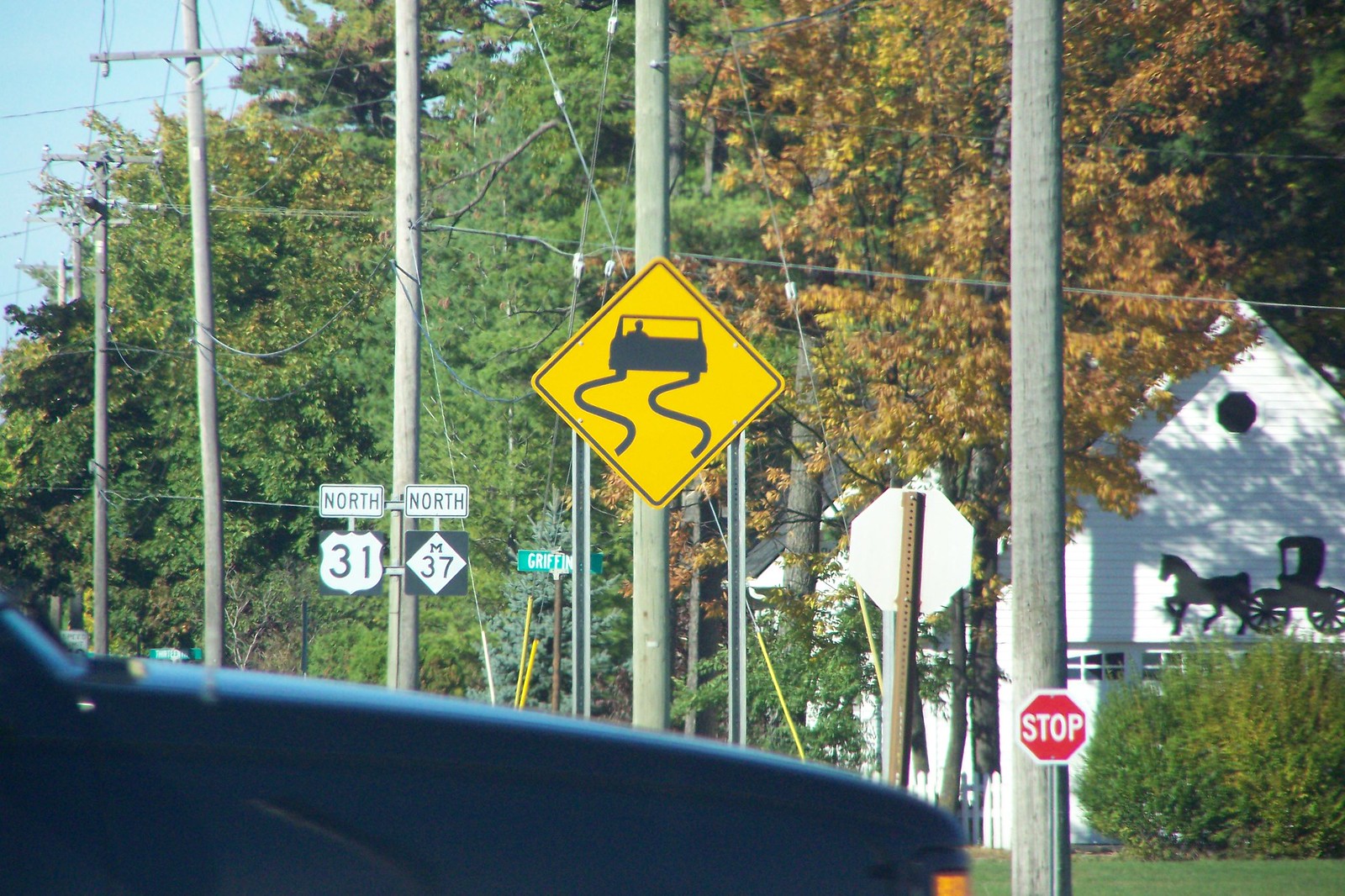This outdoor, rectangular photograph stretches slightly wider than its height, capturing a verdant landscape with a blend of autumn and evergreen trees. In the upper left corner, a bit of blue sky peeks through amidst the dense foliage. The trees span the entire background, with one tree on the far right boasting faded fall colors while the remaining trees are lush and green, possibly evergreens. Stretching diagonally from right to left are six telephone poles, diminishing in size as they recede into the distance. The first telephone pole on the right features a small stop sign at its base, while a street sign indicating Route 31 and 37 is visible on the left. In the lower left corner, a slightly out-of-focus vehicle, possibly a truck or car, intrudes into the frame, showing just the front part and a bit of the top.